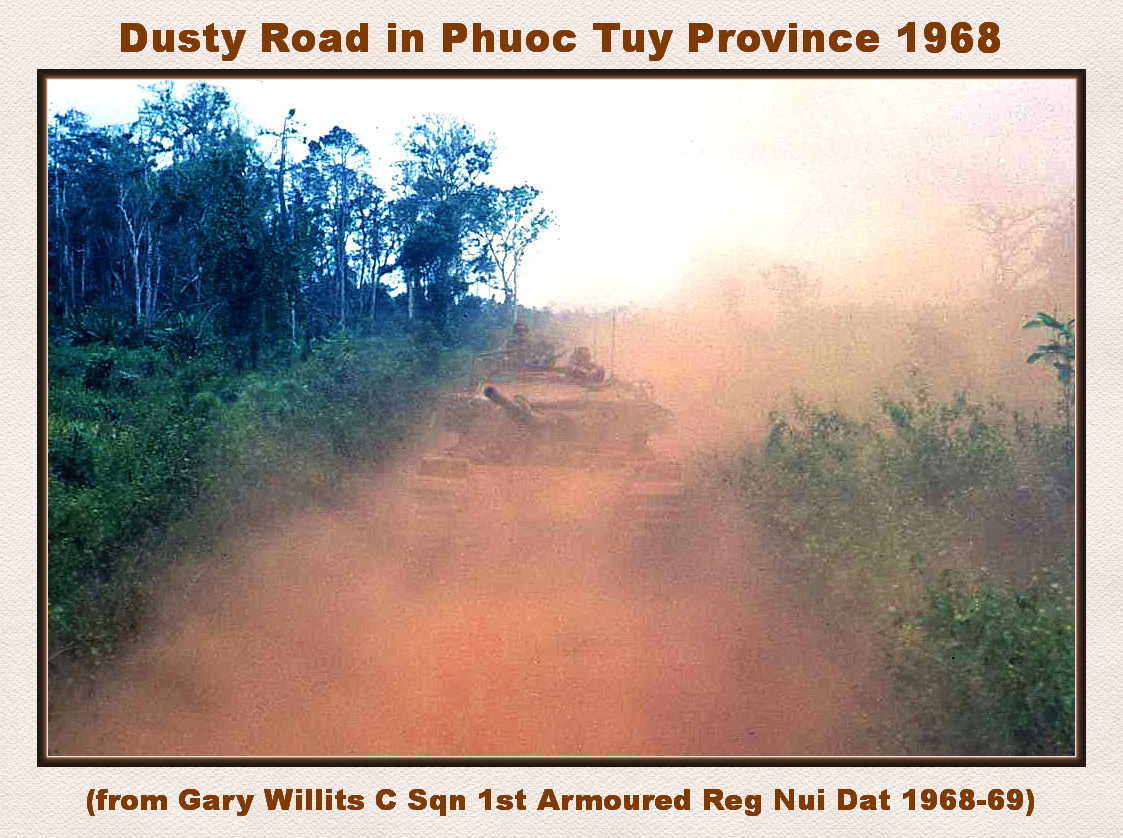The image depicts a military tank advancing down a dusty, red dirt road in Vietnam, specifically in Phuoc Tuy Province, 1968. The photograph is enclosed in a grainy, white, textured frame reminiscent of paper with a dark, almost gold inset separating the image from the border. At the top of the frame, in dark orange-red text, the caption reads, "Dusty Road in Phuoc Tuy Province, 1968." Beneath the photograph, in smaller text of the same color, it states, "(From Gary Willett's Sea Squadron, 1st Armored Regiment, Nui Dat, 1968-1969)." The tank, slightly obscured by the red dust it kicks up, is centered in the image, with its gun pointing towards the viewer. Two or three soldiers are faintly visible atop the tank through the haze. On both sides of the road, there's vegetation: green foliage on the left, including a group of trees in the top-left corner, and dust-covered bushes and scrubby trees on the right. The sky overhead is grey, indicating daylight without direct sunlight. The photo captures a stark, momentous scene from the Vietnam War, framed in a postal card-like design.